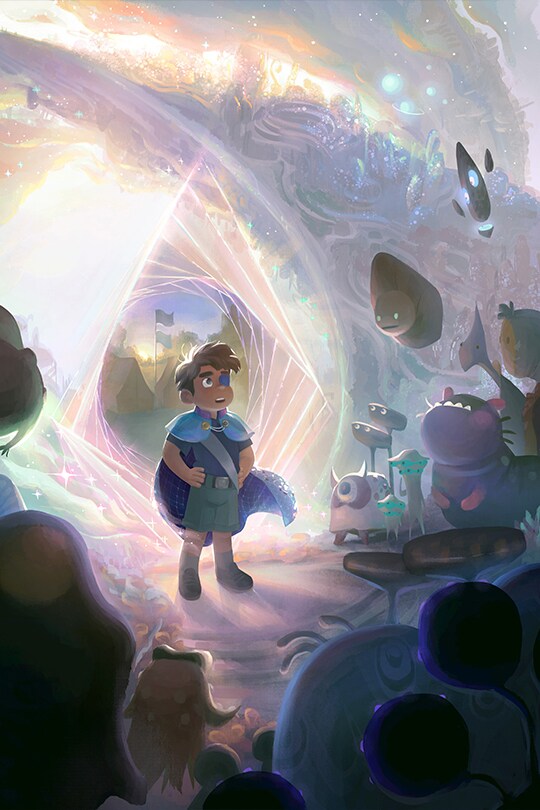In this vibrant, cartoon-style artwork or animation, a young boy, who appears to have entered a magical realm through a shimmering portal, stands at the center. The scene is incredibly colorful and fantastical, with an iridescent, dreamy atmosphere filled with sparkly clouds in hues of purple, blue, pink, orange, white, and other pastel shades. The boy, with brown skin and brown hair, is dressed in a cape draped over his shoulder, along with a shirt, shorts, boots, and notably, a blue eyepatch over one eye. Surrounding him are a variety of otherworldly creatures that evoke a Pixar-like charm; some resemble aliens with unique features like a single large eye, while others have dinosaur-like qualities. These friendly creatures, in an array of vivid colors, appear to greet him warmly. In the background, faded flags can be seen, adding to the whimsical ambiance of this enchanting scene. There is no text present in the image.